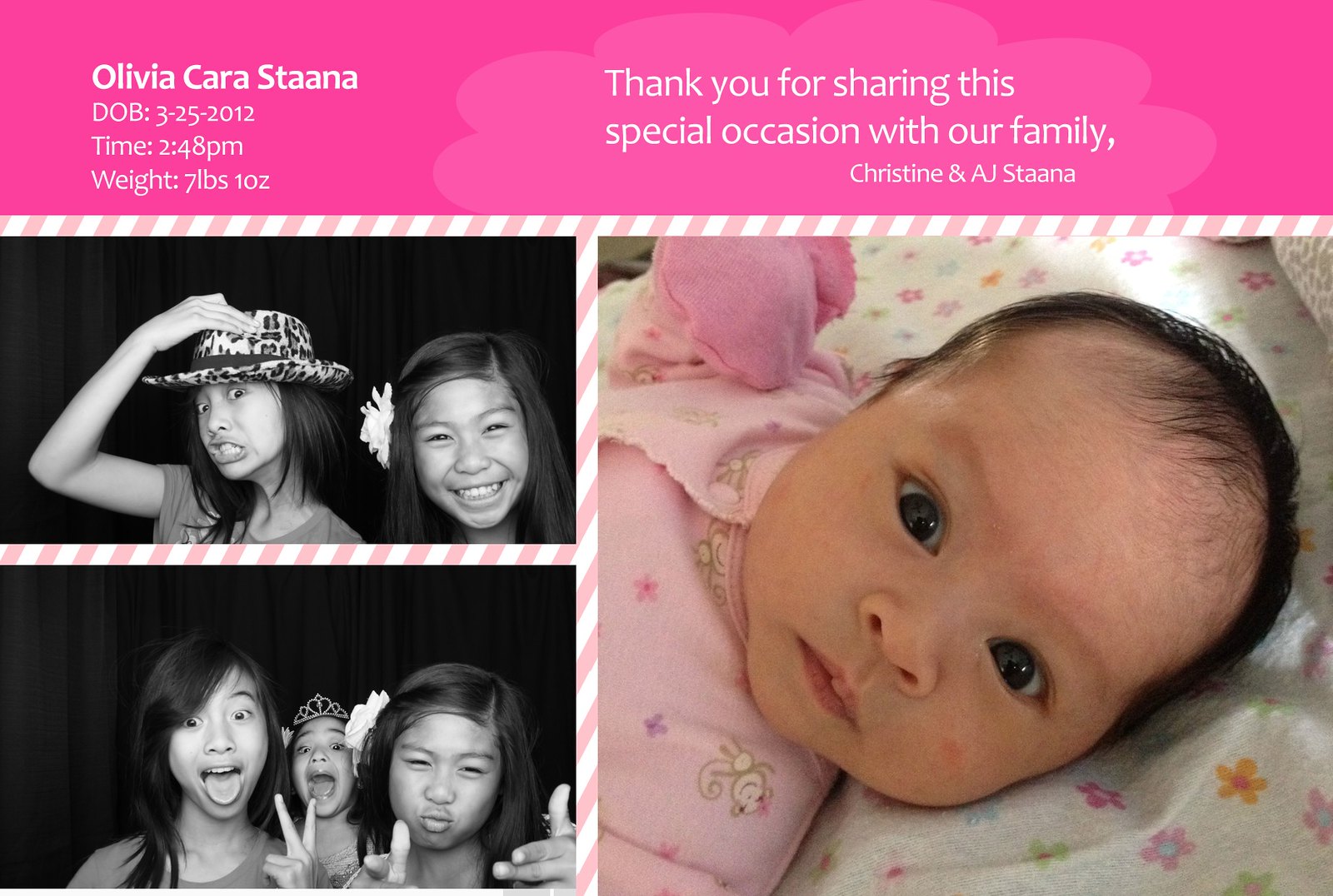Introducing the joyful arrival of Olivia Cara Stahna, this baby announcement postcard features a sweet blend of photos and heartfelt messages. Set against a vivid pink backdrop, a lightly shaded white cloud banner at the top reads: "Thank you for sharing this special occasion with our family – Christine and AJ Stahna." Beneath, in prominent white text, are the vital details: "Olivia Cara Stahna, DOB: 3-25-2012, Time: 2:48 p.m., Weight: 7 pounds 10 ounces."

Dominating the right half of the card is a tender, color photo of baby Olivia. Her wide-eyed gaze, framed by dark hair, captures the viewer’s attention. She wears a pink cotton onesie, with a matching hand glove, and lies on a white floral blanket. Though not smiling, Olivia’s curious expression is beautifully highlighted as she looks directly at the camera.

On the left, two black-and-white photo booth-style images showcase moments of amusement and affection among three young, long-haired girls. The top image features two girls: the one on the left wears a leopard print fedora while the one on the right, possibly her sister, beams a radiant smile with a flower adorning her hair. Both are in short-sleeved shirts. Below it, the three girls reappear; now hatless, the girl on the left playfully sticks out her tongue and flashes a peace sign. The girl on the right strikes a humorous, cool pose, lips pursed "Zoolander" style, with finger guns aimed at the camera, while the middle girl wears a tiara, her mouth wide open as if she’s shouting in delight.

This beautifully crafted card encapsulates the joy and excitement surrounding Olivia’s birth, commemorated with love and shared with the warmth of family and friends.